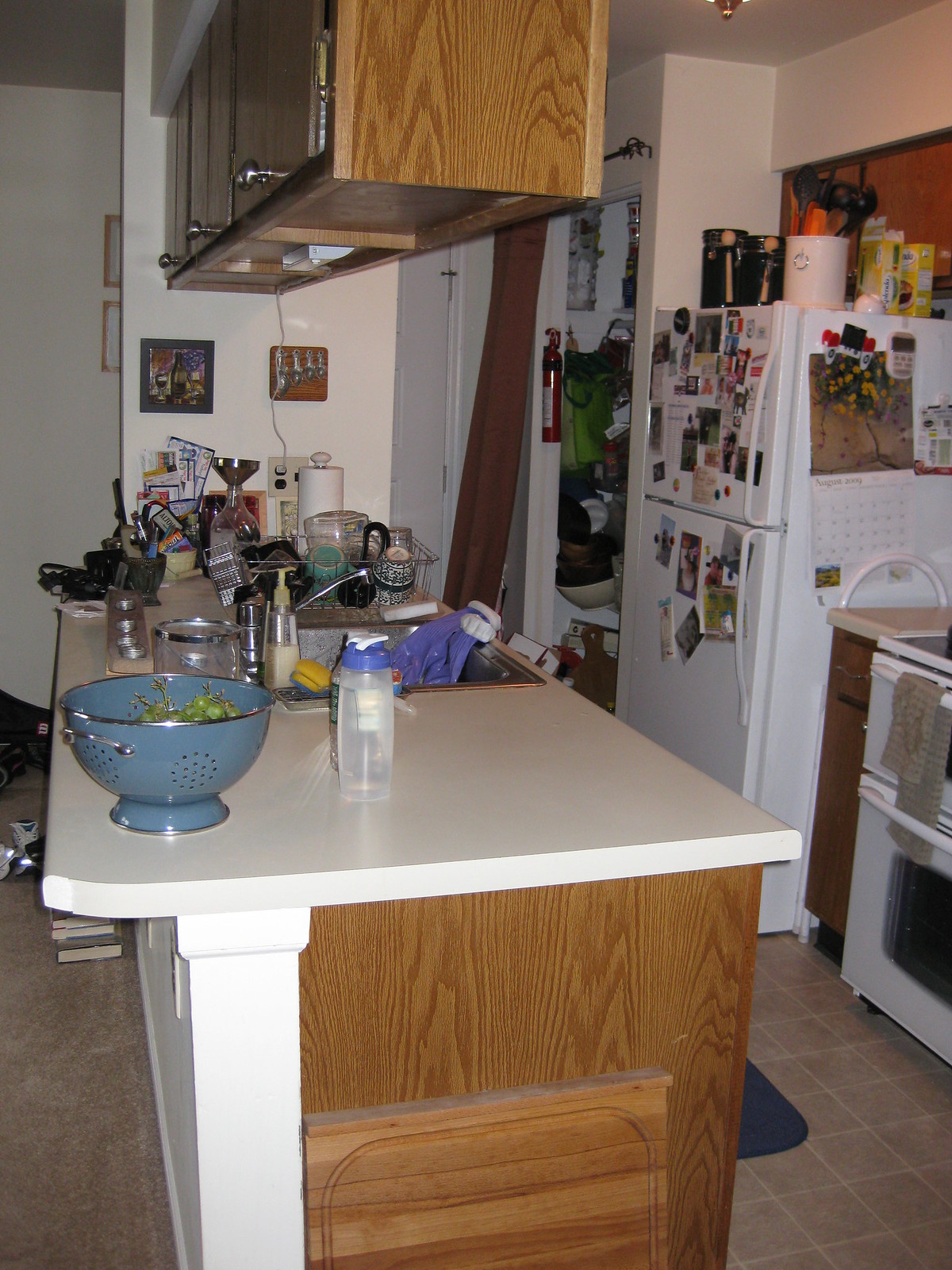Indoor color photograph capturing a cluttered kitchen scene. The image is taken from a viewpoint that includes a kitchen galley on the right side, and a central kitchen island that extends from the foreground to the background, separating the kitchen from an adjacent space that appears to be the dining room, which is out of frame to the left.

The kitchen countertop is white, likely made of simple linoleum, and its edge is finished with plywood. The countertop itself is cluttered with various cooking items. In the foreground to the left, a blue salad bowl filled with green grapes can be seen. To the right of the bowl, there is a water bottle with a blue cap. Further to the right, near the edge of the countertop, is a stainless steel sink with a strainer beside it, which is filled with various items.

In the upper left corner, kitchen cabinets are partially visible, extending into the frame. On the far right edge of the image, part of an oven door can be seen. Positioned further back, a white refrigerator stands loaded with pictures on both the freezer door at the top and the refrigerator door at the bottom. The top of the refrigerator holds additional clutter.

In the background, to the left of the refrigerator, an open linen closet or pantry door reveals more clutter inside. The kitchen floor, visible in the lower right corner, is composed of square, brown tiles, while on the other side of the island, light brown carpeting is visible, suggesting the transition to the dining room or living area. The photograph contains no legible text or print.